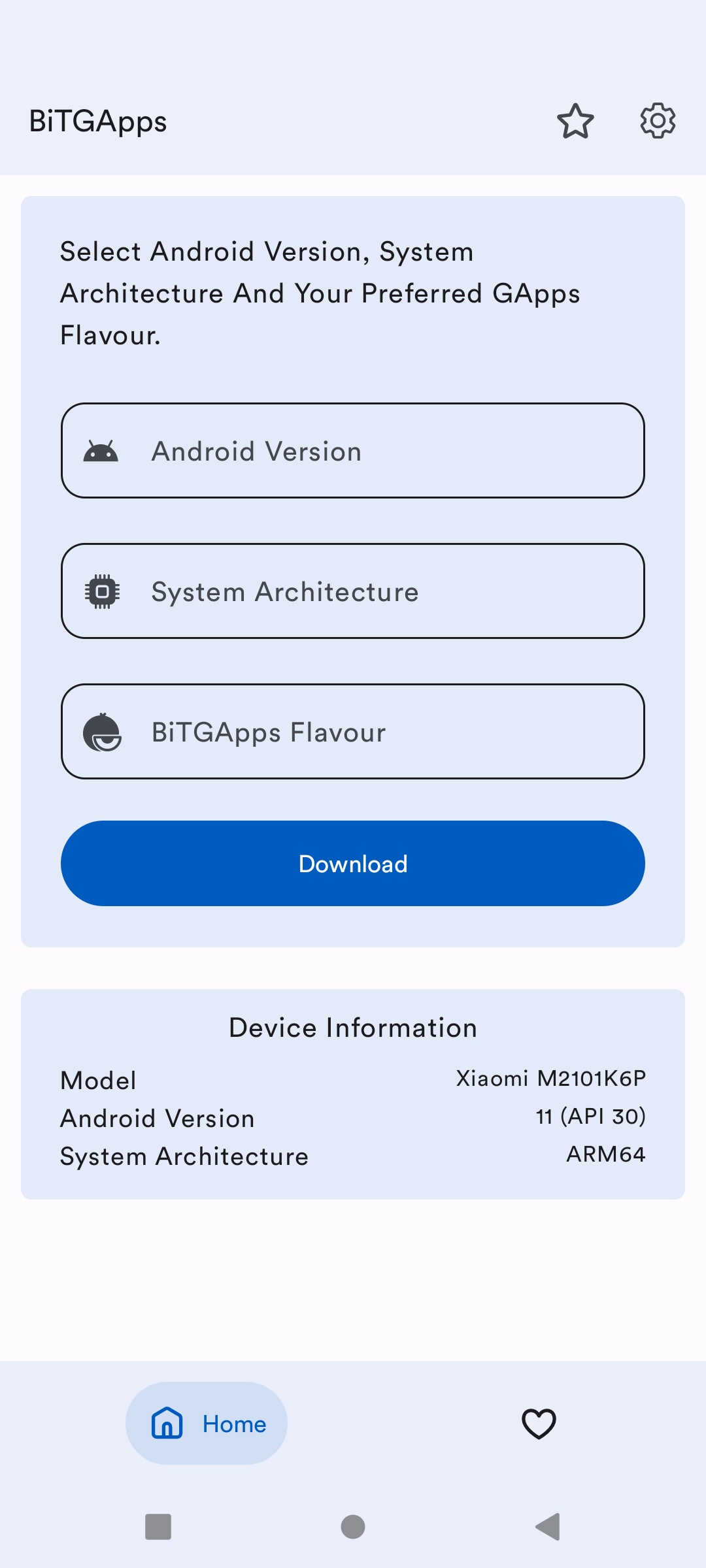At the top of the image, the background is entirely gray. On the left side, various pieces of text are visible, including "BITGA, BPS, holo.star, gear." Additional captions read "gray," "select Android version," "system architecture," and "your preferred apps flavor." 

Towards the middle of the image, there's an oval labeled "Android version." More centered text reads "system architecture," with a tips section to the left. There is also a rounded section featuring what looks like a fruit, possibly a melon, labeled "BITG apps flavor."

The image contains blue text displaying device information such as "Model: Xiaomi M2-101K6P," "Android version: 11," "API: 30," and "system architecture: ARM64." Below this is a white bar, followed by more gray sections, including an oval that says "home." There are icons such as a holo.heart, a gray square, a circle, and a left arrow.

This screen appears to be related to BITG apps on a Xiaomi smartphone, emphasizing different visual elements like backgrounds, borders, and lettering, which are somewhat out of focus around the edges. The elements "home," "heart," "square," "circle," and "left arrow" provide navigation functions within this interface.